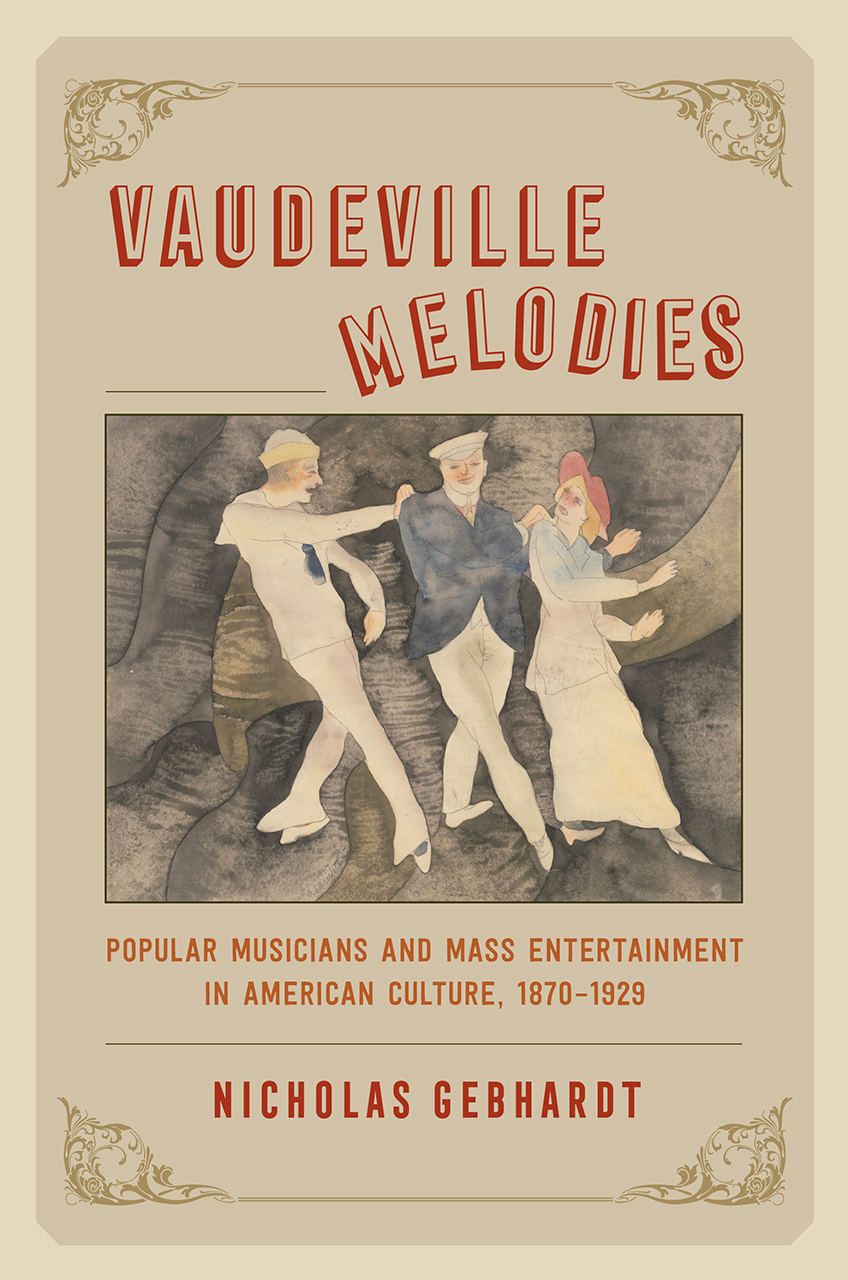This image depicts the cover of a book or vintage pamphlet titled "VAUDEVILLE MELODIES," designed in an elaborate and artistic style. The cover is vertically rectangular with a gray border and a darker gray background, complemented by gold decorative scrolls in each of the four corners, connected by gold lines at the top and bottom. 

The title "VAUDEVILLE MELODIES" is prominently displayed at the top in bold, uppercase red letters. Below the title, there is a watercolor painting featuring three figures—a woman in a blue dress with a red hat, and two men, one of whom is wearing a blue suit jacket, while the central figure appears to be donning a sailor's cap. These figures are depicted in mid-dance, evoking the lively spirit of vaudeville entertainment.

Beneath the painting, in orange, is the text: "Popular Musicians and Mass Entertainment in American Culture from 1870 to 1929." The author's name, "Nicholas GEBHARDT," is prominently displayed in bold red letters below the subtitle. This cover art, with its vintage aesthetic and detailed illustration, captures the essence of American cultural entertainment history.